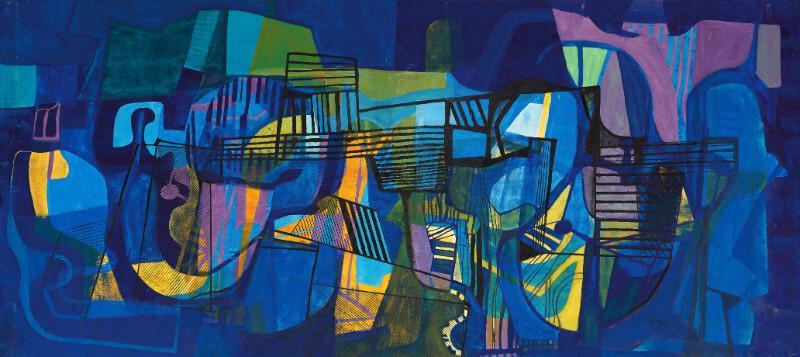This image features a striking abstract painting characterized by its rich and varied color palette. The painting is a horizontal rectangle, approximately two and a half times as wide as it is tall. Dominated by a deep, rich blue, the artwork encompasses a wide spectrum of colors, including yellow, orange, purple, green, light green, and pink. These colors form an array of shapes and patterns, both geometric and freeform, without depicting any specific recognizable objects.

The painting features an intricate interplay of lines and shapes: there are diagonal, horizontal, and vertical black lines crisscrossing the canvas, contributing to the dynamic, almost graffiti-like texture, especially in the center where it hints at indistinct graffiti text in yellows and pinks. In the upper right corner, a pinkish shape resembles an abstract bird with its wings spread, adding an element of intrigue. To the far left, a yellow figure appears, suggestive of a bird or duck's head adorned with what looks like a black hat outlined in pink. This detailed use of color and form creates a jazzy, vivid piece that remains true to its abstract nature, inviting viewers to delve into their interpretations.